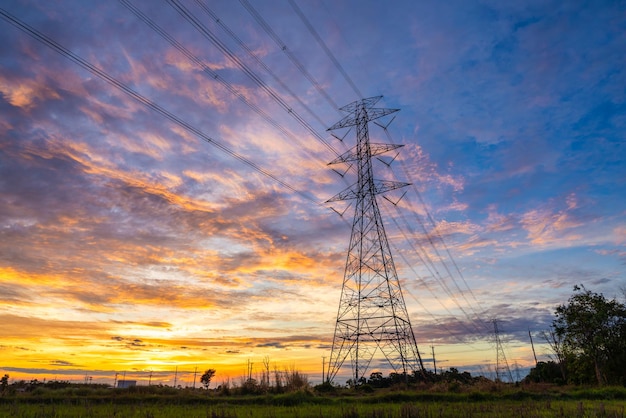This photograph showcases a striking landscape at either sunrise or sunset, featuring a large, imposing power line tower with numerous heavy-duty electrical lines extending into the distance. The metal structure, standing approximately 50 feet tall with multiple arms supporting six to eight power lines, is set against a stunning sky painted with gold, pink, orange, and blue hues, which reflect off scattered clouds near the horizon. In the background, you can spot a distant power line tower and the silhouettes of buildings on the skyline, suggesting a semi-rural area. The scene is dotted with a few trees, adding a touch of nature to this otherwise industrial vista.